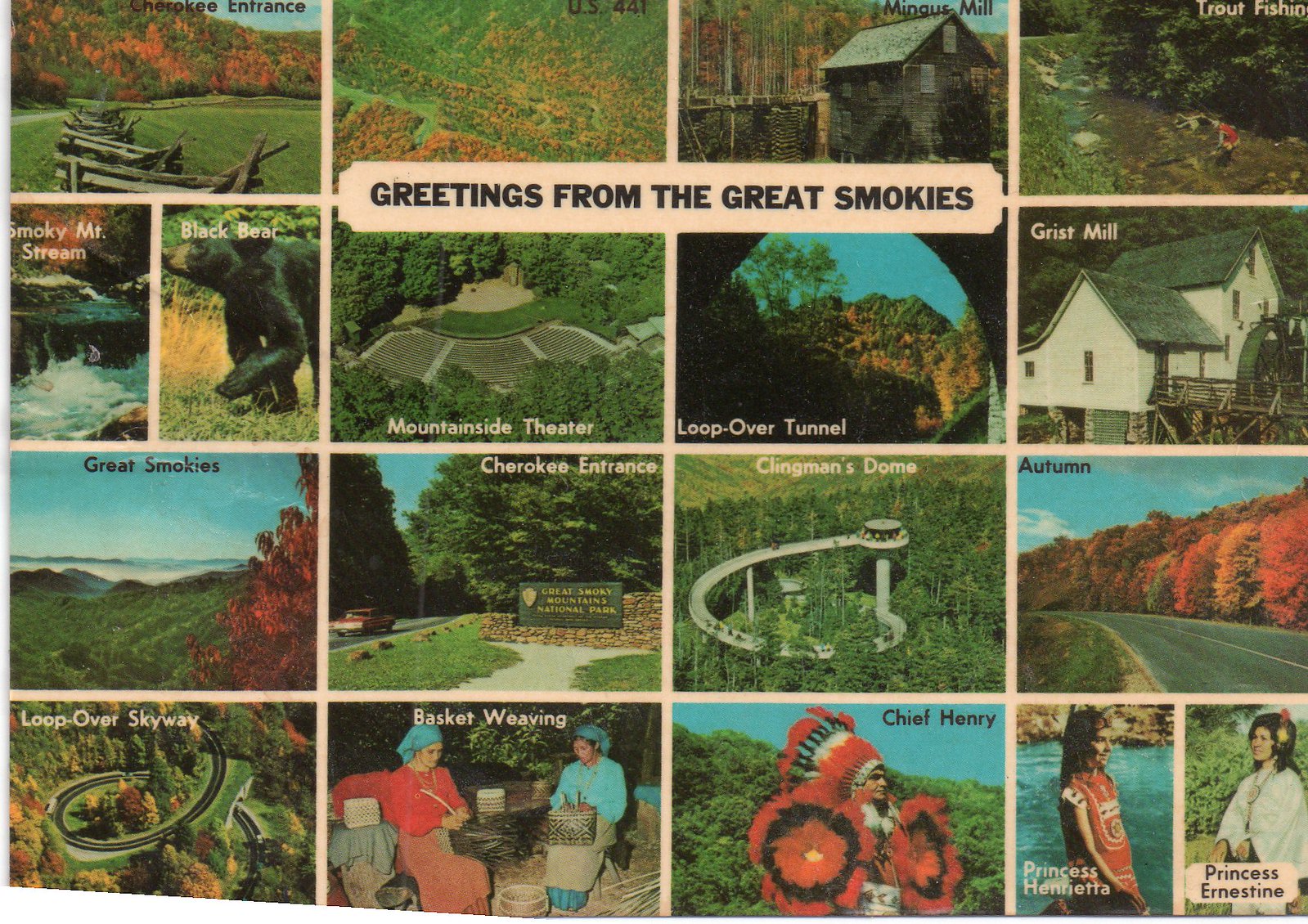This image appears to be a vintage postcard with the title "Greetings from the Great Smokies" prominently displayed at the top. The postcard features a 4x4 grid of various photographs showcasing key attractions and scenes from the Great Smoky Mountains National Park. Starting from the top left and moving right, the first image captures the Cherokee Entrance along US 441, featuring lush, green grass and possibly some wood or firewood. The next images include Mingus Mill and a scene depicting trout fishing. In the second row, photos feature a Smoky Mountain Stream, a photograph of a black bear labeled "Black Bear," the Mountainside Theater, the Loopover Tunnel, and another grist mill. The third row offers a scenic view from a mountain top with the label "Great Smokies," another shot of the Cherokee Entrance, the intriguing Clingmans Dome with its circular ramp, and an autumn landscape. The final row displays cultural elements: the Loopover Skyway, people engaged in basket weaving, a photograph of Chief Henry, and portraits of Princess Henrietta and Princess Ernestine. The postcard gives a rich visual tour of natural landscapes, wildlife, rustic buildings, and cultural heritage associated with the Great Smoky Mountains.